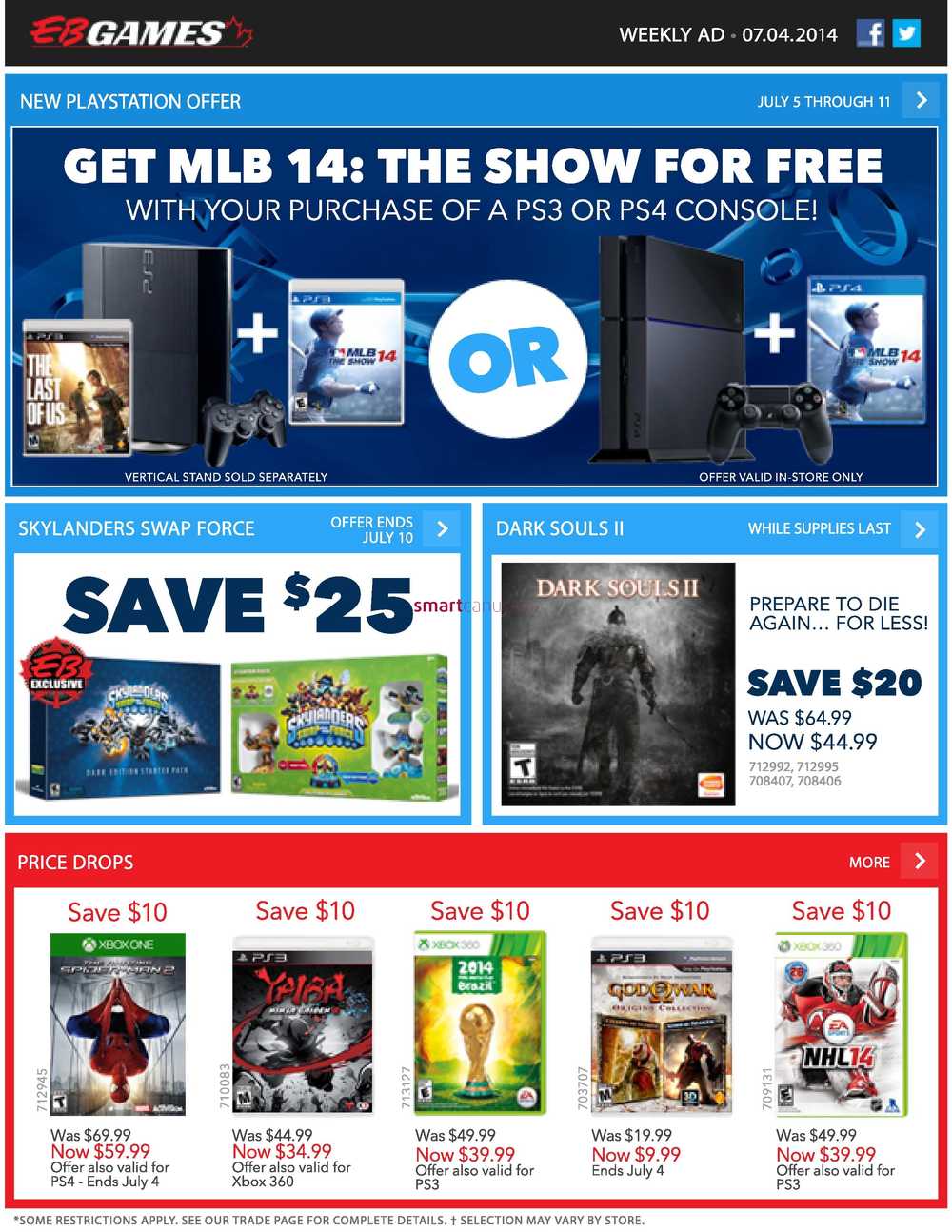**Title:** Weekly Ad for EB Games (July 4, 2014)

**Description:**

This vibrant advertisement from EB Games, predominantly featuring a blue color scheme, showcases a variety of gaming deals and promotions for the week of July 4, 2014. 

At the forefront, there is a special offer for PlayStation enthusiasts: purchase a PS3 or PS4 console and receive a complimentary copy of "MLB 14: The Show." The promotion is visually emphasized with images of both PS3 and PS4 consoles accompanied by controllers, each featuring the MLB game.

Below this, a separate ad highlights a limited-time offer ending on July 10, 2014. Shoppers can save $25 on two Skylanders games—one of which is depicted in blue, while the other appears to showcase action figures.

Additionally, there are markdowns on several other popular games, available while supplies last:
- **Dark Souls 2: Prepare to Die Again Edition** – Save $20, now priced at $44.99 (previously $64.99).
- **The Amazing Spider-Man 2** for Xbox One – Save $10, now $59.99 (previously $69.99).
- **Yarya** for Xbox One – Save $10, now $34.99 (previously $44.99).
- **FIFA World Cup Brazil 2014** – Save $10, now $39.99 (previously $49.99), available for both Xbox 360 and PS3.
- **God of War** – Save $1, now $9.99 (previously $10.99), valid until July 4, 2014.
- **NHL 14** – Save $10, now $39.99 (previously $49.99), for both Xbox 360 and PS3.

The ad also includes links to EB Games' social media accounts on Facebook and Twitter, encouraging customers to stay connected for future updates and promotions.